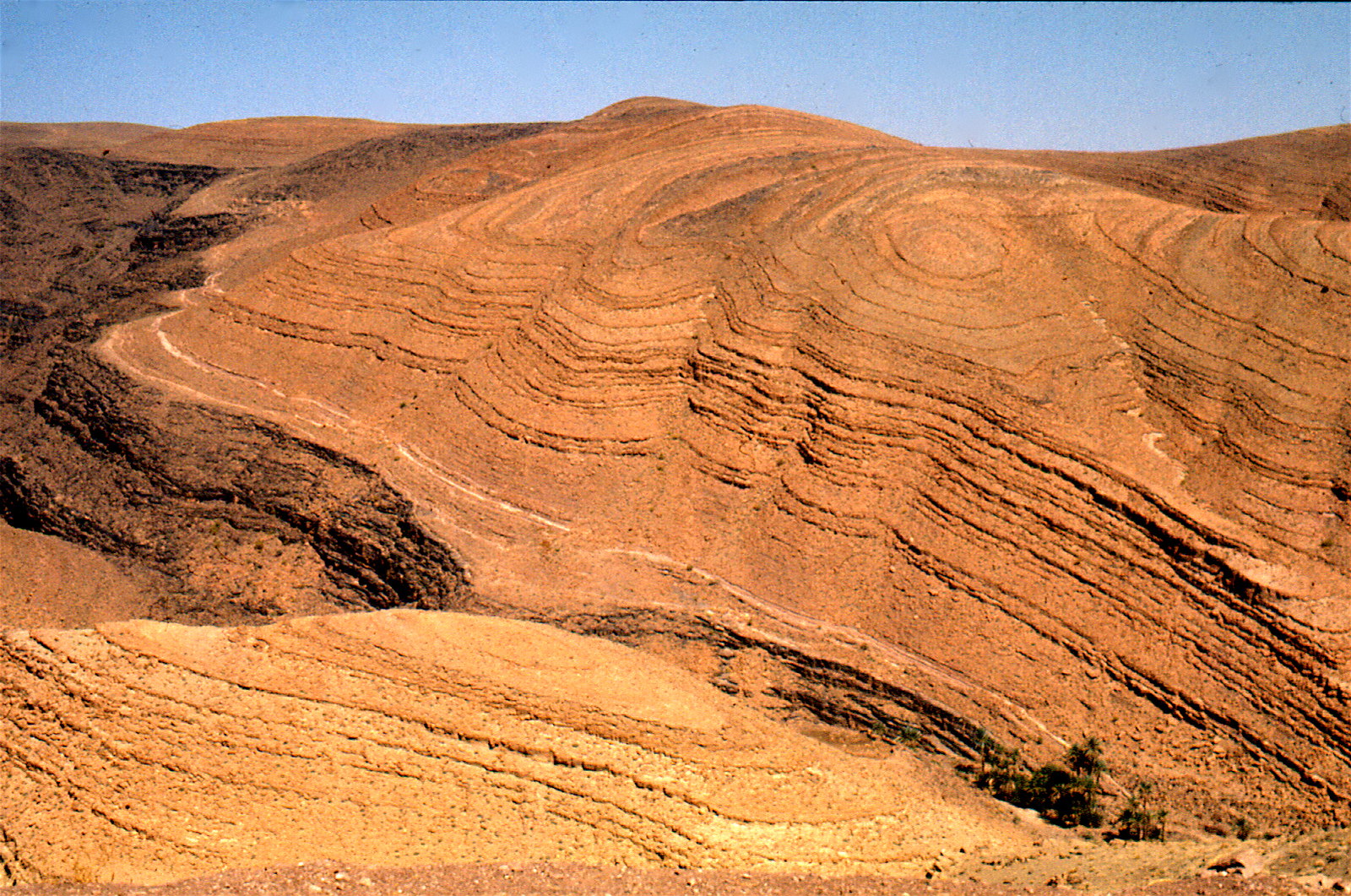The photograph captures a striking desert landscape dominated by reddish-orange and yellowish-orange rocky terrain. The landscape features layers of scalloped, rocky formations that give it a distinct texture, suggesting the presence of either red clay or red rock mountains. The sky covers only the top seventh of the image, presenting a clear, light blue color that contrasts sharply with the arid earth below. Towards the lower right corner, there is a cluster of 12-15 palm trees forming a small oasis, accompanied by a road that winds through the rugged landscape. Darker dirt surrounds the lighter patches of sand or rock, adding depth and variation to the scene. The image may have been slightly edited, as elements appear somewhat out of focus. Overall, the photograph vividly showcases the dry, barren beauty of the desert expanse.